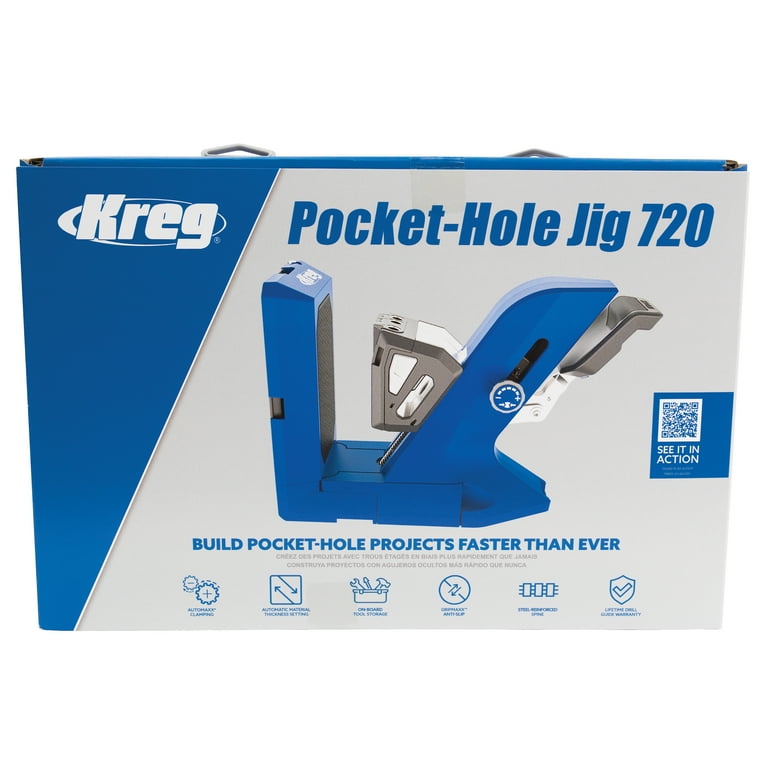This horizontal photograph showcases the packaging of the Kreg Pocket-Hole Jig 720. The centerpiece of the box features an image of the jig itself, which is a vivid blue with gleaming chrome attachments, resembling the upper part of a capital letter "K." On the right side of the packaging, there's a blue square with white lettering prompting viewers to "See it in action" accompanied by a QR code. Below the image of the jig, bold text proclaims, "Build pocket-hole projects faster than ever." Several blue-outlined symbols can be seen beneath this text. A striking blue triangular shape runs diagonally along the entire left side of the box, showcasing the manufacturer's name, Kreg, in crisp white letters within an oval. The latches on the top of the box are notably chrome-plated, adding a touch of sleekness to the overall design.